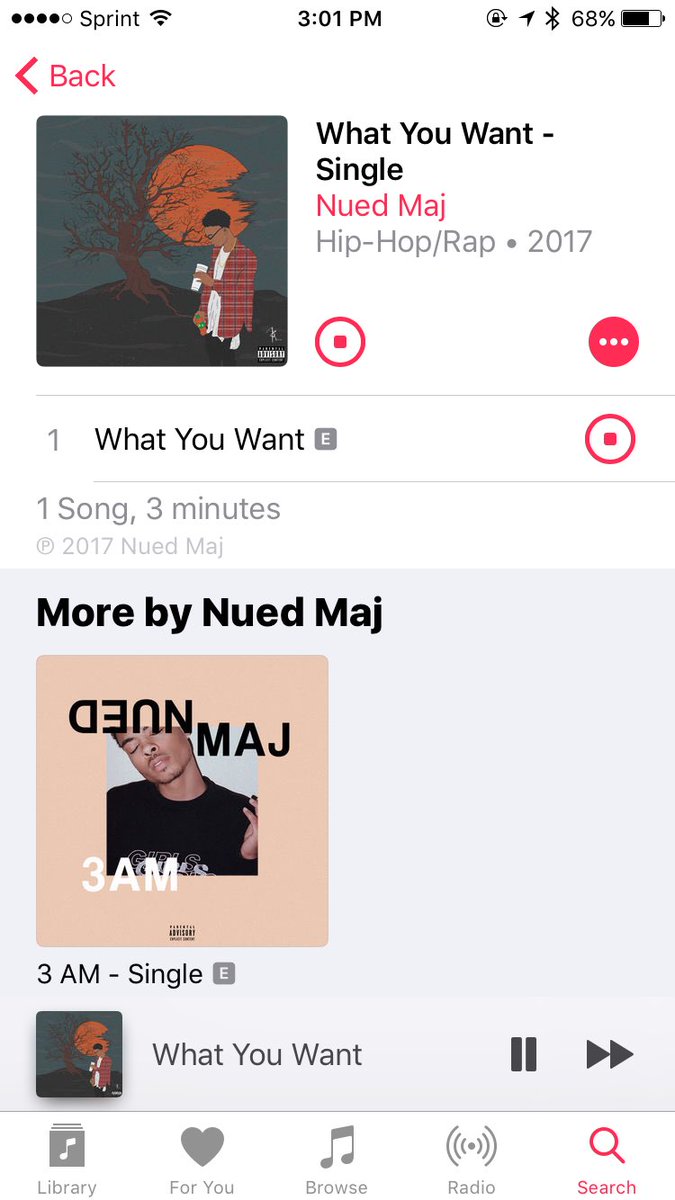Screenshot of a smartphone display captured at 3:01 p.m. with the battery level at 68%. The music player is actively running, featuring the song "What You Want" by New Ed Maj. The album art for the song is prominently displayed as a comic-style illustration of a melancholic man under an orange moon in a leafless autumn setting. The genre is classified as Hip-Hop/Rap, released in 2017. The player interface shows Pause, and Fast Forward controls, with the song's duration listed as 3 minutes. Additionally, an image of the artist New Ed Maj is shown wearing a black shirt and posing with his left hand up, head tilted slightly, while his name appears in mirror image on the graphic. Another single titled "3 A.M." by the same artist is also noted on the screen. However, the exact progress through the song "What You Want" is not indicated.